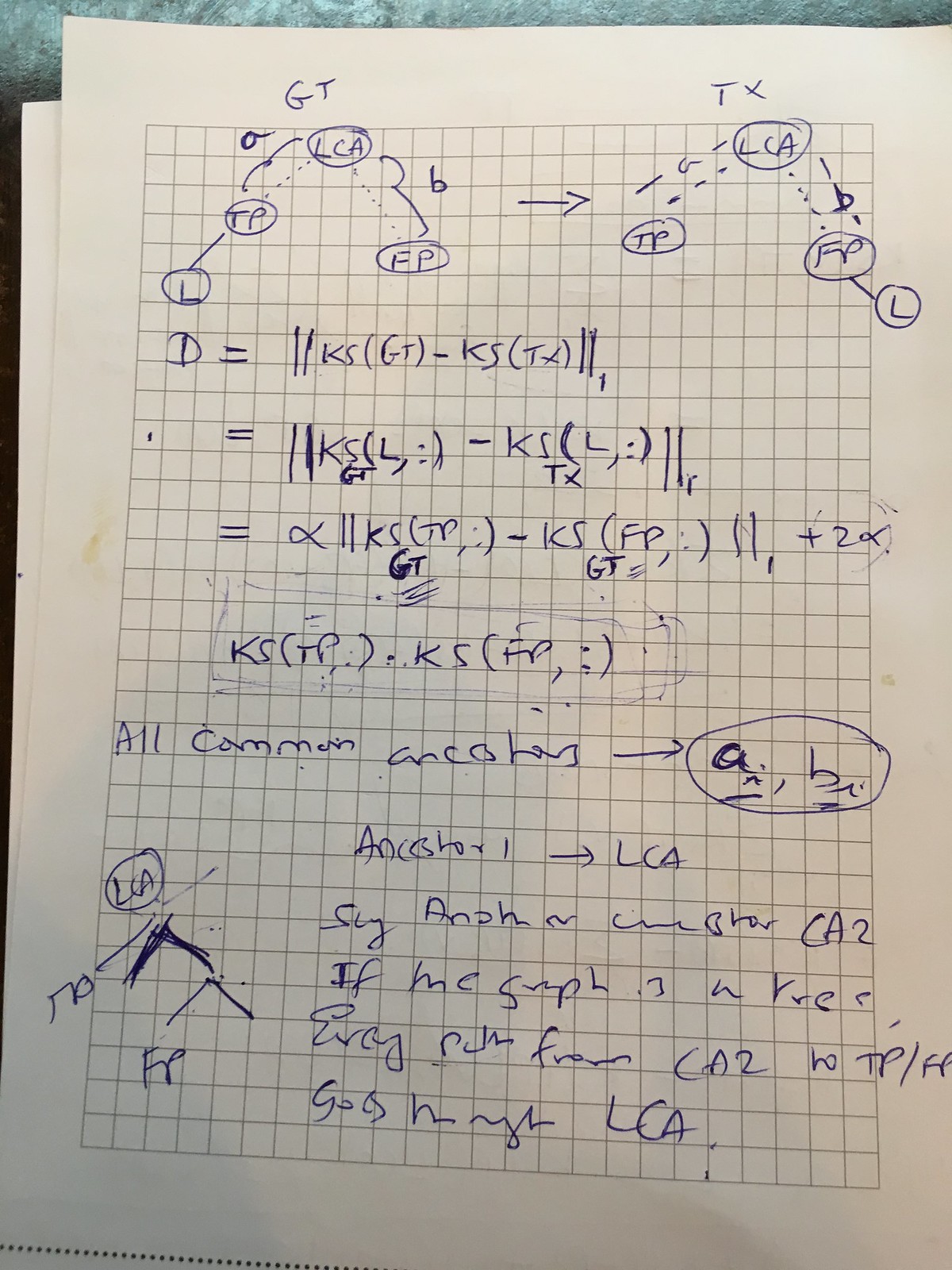The image depicts a detailed worksheet on a standard white sheet of paper, featuring faintly drawn grid lines in pale gray. The worksheet is filled with various graphs, equations, and annotations that suggest calculations related to ancestry. In the center of the page, the phrase "All Common Ancestors A, B" is prominently displayed, with 'A' and 'B' encircled for emphasis. Below this, there is an indication of "Ancestor 1" followed by an arrow pointing to "LCA." Despite the handwriting being somewhat challenging to decipher, key phrases such as "if the tree graph is a tree," "LCA," "CA2," and "TP & FP" can still be discerned. Additional graphs and arrows further illustrate the connections between elements such as "L" to "TP" and "LCA" to "FP," offering a visual representation of the ancestral relationships being analyzed.